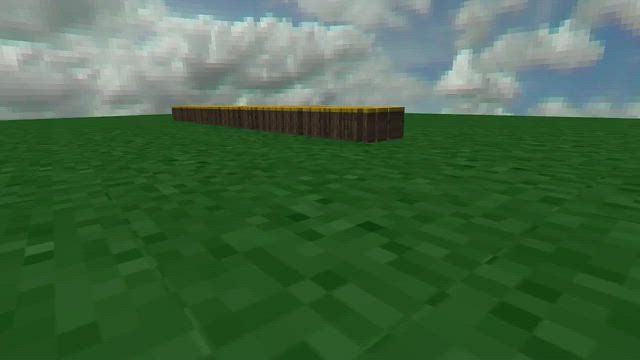A computer-rendered image reminiscent of classic video games features a highly pixelated and blocky aesthetic. Dominating the scene is a landscape of green grass, presented in distinct, chunky blocks. Above, a blue sky is depicted in a similarly pixelated style, dotted with block-shaped clouds. Central to the image is a long, brown structure with a somewhat distressed appearance, punctuated by lighter, whitish areas. Atop this structure sits a yellowish element, enhancing the retro, pixelated charm of the scene. The entire composition evokes a nostalgic, old-school video game ambiance.